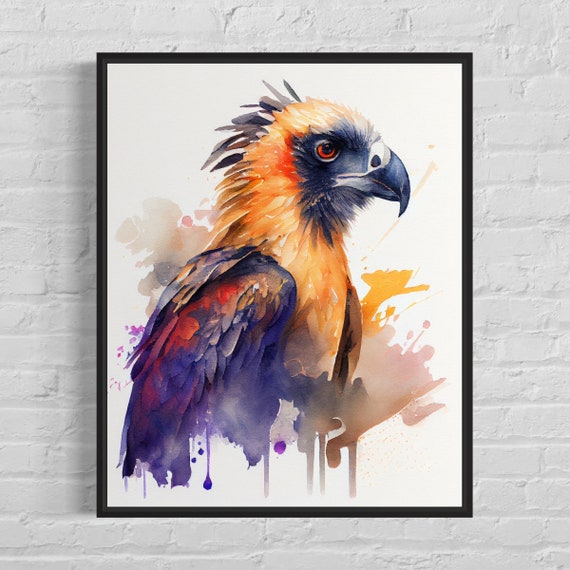The image depicts a watercolor painting of a vibrant, fantastical bird that resembles a hawk but features an array of non-traditional, striking colors. The bird, shown in side profile facing the right, is surrounded by a white background accented with splashes of pink, peach, gray, and black. This artwork is mounted within a thin black frame and hangs centrally on a light gray, white-painted brick wall, suggesting it could be in a room or possibly a museum setting. The bird itself is adorned with a spectacular mix of colors: the beak is black, the eyes are red, and the feathers around the eyes and chin are dark. The feathers from the top of the head down to the breast are an orangish-yellow, while those on the back of the head darken. The wing feathers display a stunning gradient of dark blue, red, purplish, pink, and light blue hues. Also notable are some parrot-like feathers atop its head, adding an exotic flair to its appearance.